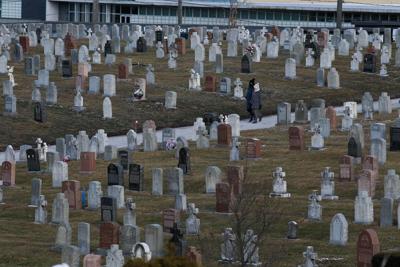The photograph captures a vast, outdoor cemetery during the daytime, showcasing a mix of gravestones of various colors and shapes. A white path runs diagonally from the mid-left to the mid-right, flanked by tombstones ranging from black, white, reddish, and gray, with shapes that include crosses, squares, and rounds. Two individuals in dark clothing and boots, with toboggans on their heads, are visible walking along this path. They appear as a couple, one dressed in all black and the other in gray. The cemetery's grass looks unhealthy, tinged with brown amidst the green, and is dotted with a few flowers placed in front of graves. A skeletal, leafless tree stands prominently in the foreground, adding to the overall dull atmosphere. In the distance, behind the fenced boundary of the cemetery, a white and black factory-like building with numerous windows looms, further contributing to the austere setting.